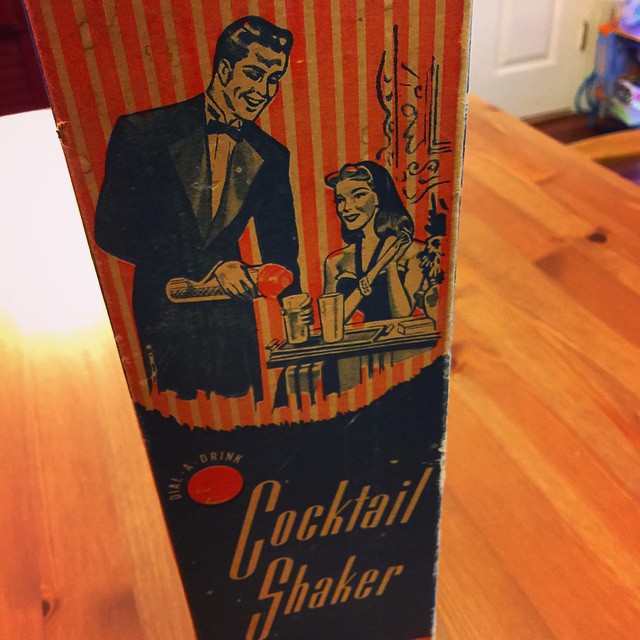This close-up photograph showcases a vintage cardboard packaging for a cocktail shaker, resting on a light brown, highly-polished wooden table. The box is a tall, rectangular shape, fitting the silhouette of a cocktail shaker. It features a black-and-white cartoon illustration of a man in a black tuxedo with a bow tie and slicked-back hair, happily pouring a drink from a metal tube into a clear glass. The glass is placed on a table where a lady in a black cocktail dress is seated, watching the man with a smile. The lower part of the packaging is black, with a large gold text that reads "Cocktail Shaker" prominently displayed. Additionally, there is a small red circle on the top left corner within the black section with the words "Dial a Drink Around It." The edges of the box appear a bit worn, adding to its vintage charm. In the background, towards the top right corner of the image, a white painted door can be seen, indicating an indoor setting.